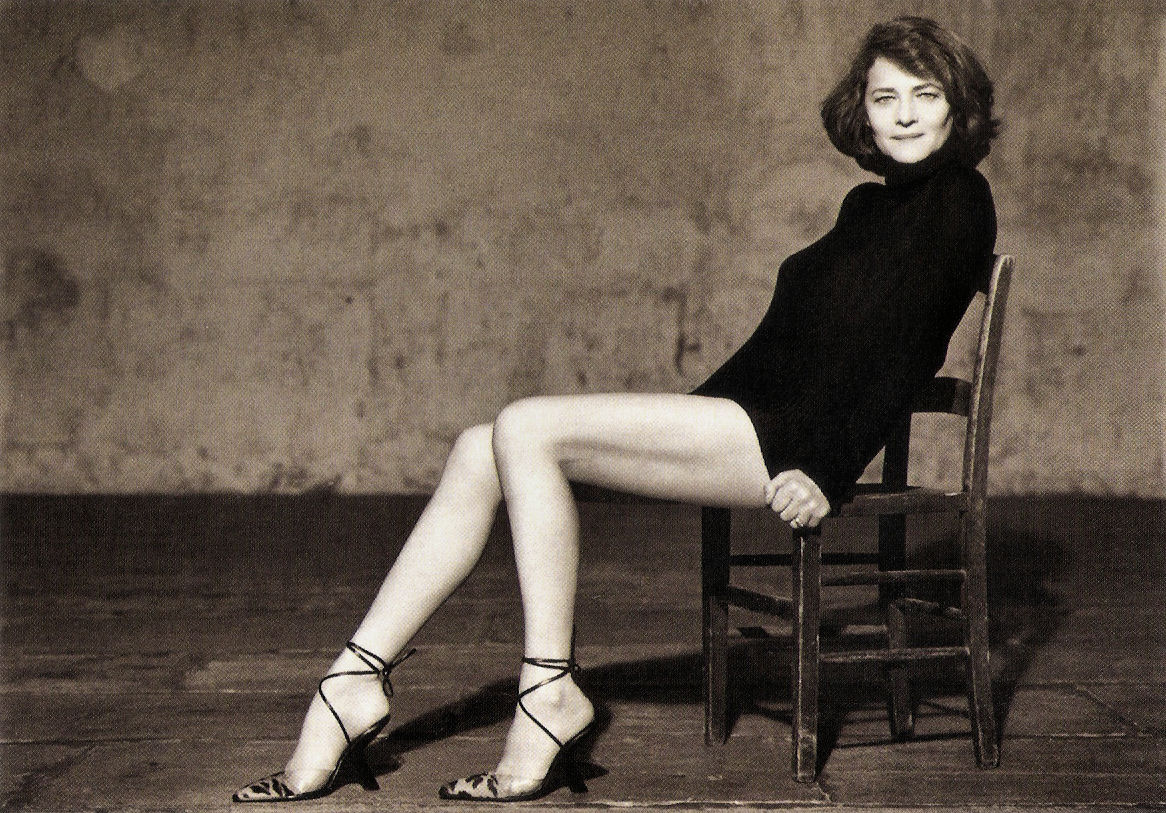The black and white photograph portrays a woman sitting on an old wooden chair with a straight back and four sturdy legs, situated in a room with grimy, aged cement walls and a wooden plank floor. The woman, with her voluminous shoulder-length hair, sits on the edge of the seat, reclining slightly. Her attire, a form-fitting bodysuit that covers her from her bottom up to her neck and arms, suggests the appearance of a short dress due to its minimal coverage over her legs, which are long and uncovered. She wears high-heeled shoes that feature a closed toe and delicate spaghetti straps wrapping around her ankles. She gazes directly at the camera with a slight smile, exuding a confident and poised demeanor. The overall ambiance of the image is vintage and somewhat stark, accentuated by the black and white tones.